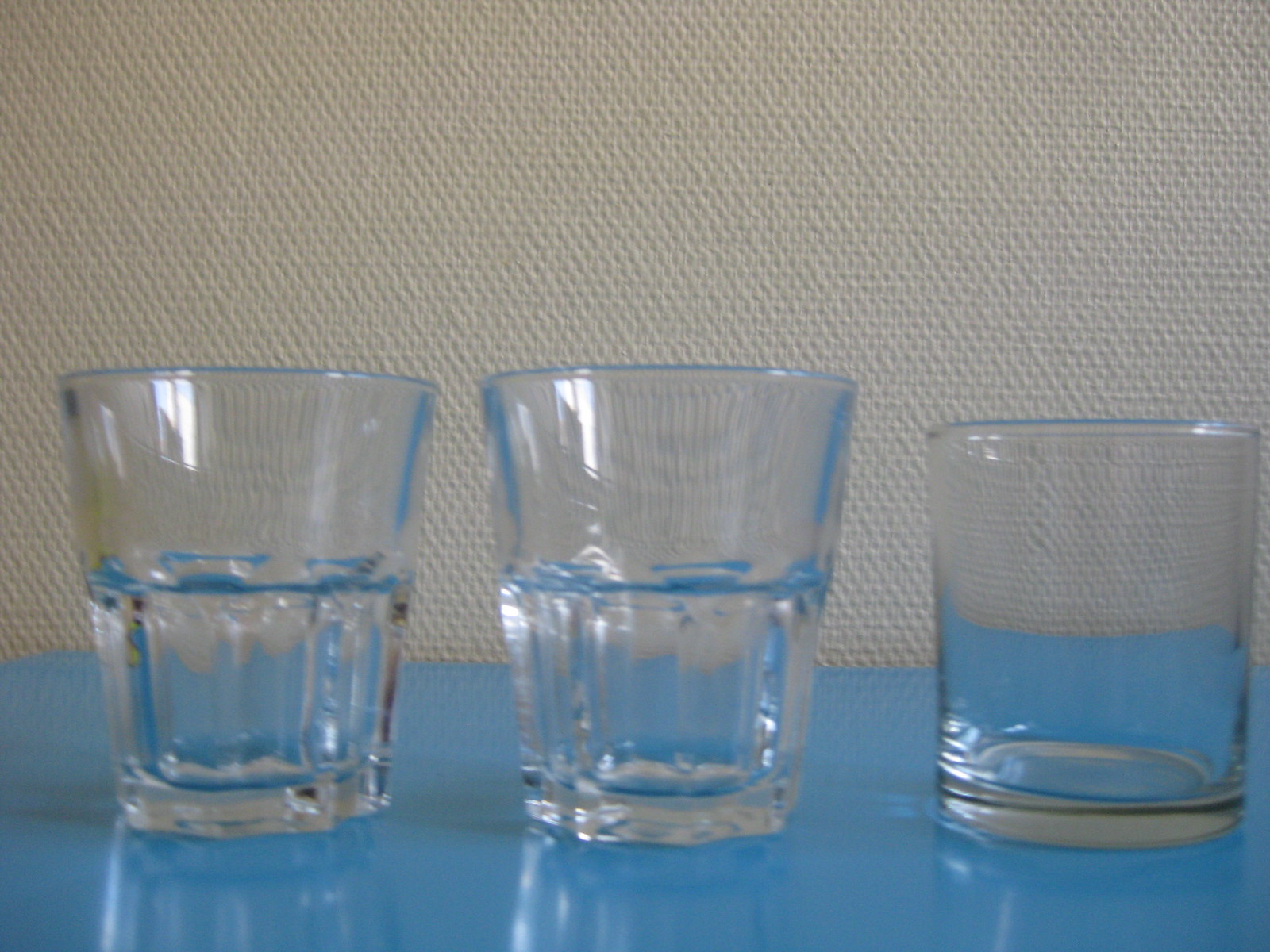In this close-up photograph, three clear shot glasses are arranged on a sky-blue, hard surface that resembles a kitchen table or countertop. The background features off-white, textured wallpaper that provides a simple, unobtrusive backdrop. Of the three glasses, the left two are identical with ridges near the bottom, a thick base, and a wide, smooth opening at the top. In contrast, the glass on the right is a plain cylindrical shape with an even thicker base, making it slightly taller and more substantial. The glasses are empty and positioned close together, nearly filling the frame without touching each other. The blue surface reflects subtly onto the clear glass, adding a delicate hue to the transparent material. The image captures about two-thirds of the shot glasses, the rest showcasing the minimalist background. The photo, though a bit blurry, highlights the detailed differences in glass design against a calm, simple backdrop.